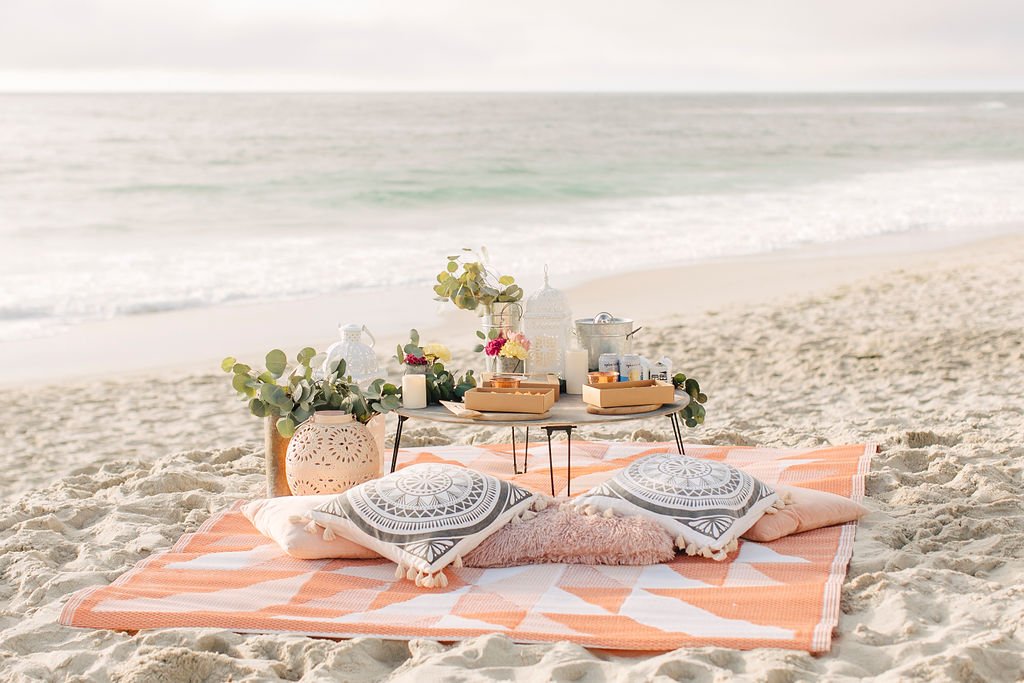This detailed image depicts an idyllic, Instagram-worthy beachside picnic set against a backdrop of a cloudy, gray sky and a serene, turquoise-green ocean with gentle, flat waves lapping onto the sandy shore. The picnic area is meticulously staged on a large rug of salmon pink and white hues, featuring a triangular checkerboard pattern. On top of this elegant rug, there are several throw pillows—some white and black with intricate, mandala-esque designs, and others in shades of pink and peach, adding a cozy yet stylish touch.

Positioned near the throw pillows is a potted plant in a pink base, its green leaves spreading out vibrantly. The setup also includes a small, round table with thin black legs and a wooden brown top. This table holds several cardboard boxes likely containing food, a metal ice bucket with shiny silver finish, a couple of beer cans, and a candle, creating a sense of casual luxury. Additional decorative elements include a clear glass vase and another metal container, both filled with green foliage, complemented by a pink rose and a yellow-petaled flower, enhancing the overall aesthetic. This picturesque arrangement exudes a sense of luxury and meticulous attention to detail, making it appear straight out of a fashion magazine or lifestyle blog.